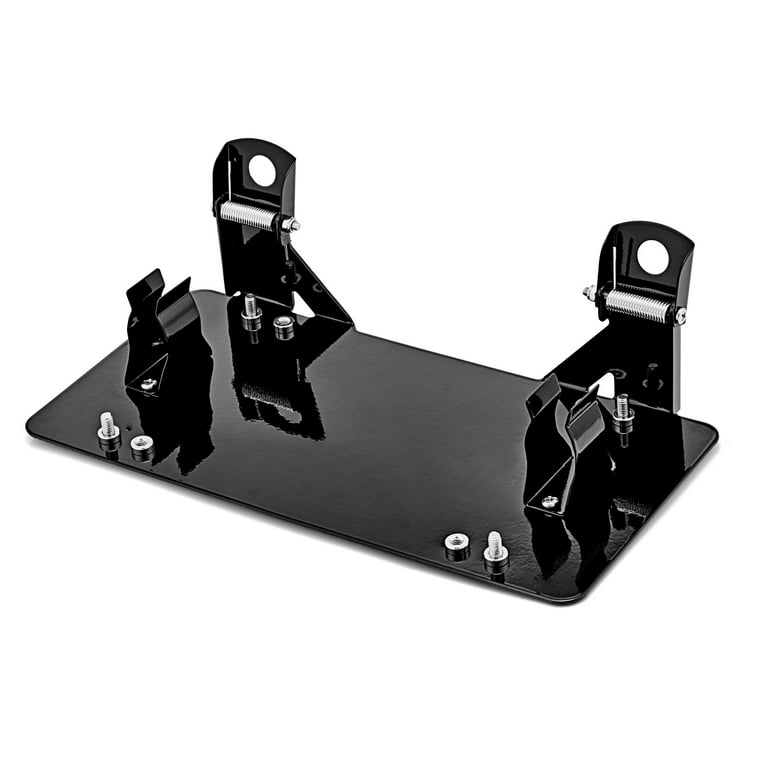This image appears to depict a sleek, shiny, flat black metal base, possibly intended for a product that could be bought on Amazon or Walmart. The base is rectangular and has several bolts and screws protruding from it. On either side of the base, there are two black metal clips or holders that might be used to secure various items such as paper, credit cards, or even a phone. Attached to the rear of the base are metal brackets that may contain springs, suggesting a potential for movement or adjustment. The overall design and the screws on top of the base resemble the mechanical structure seen in wall-mounted TV brackets, although the exact purpose of the object remains unclear.